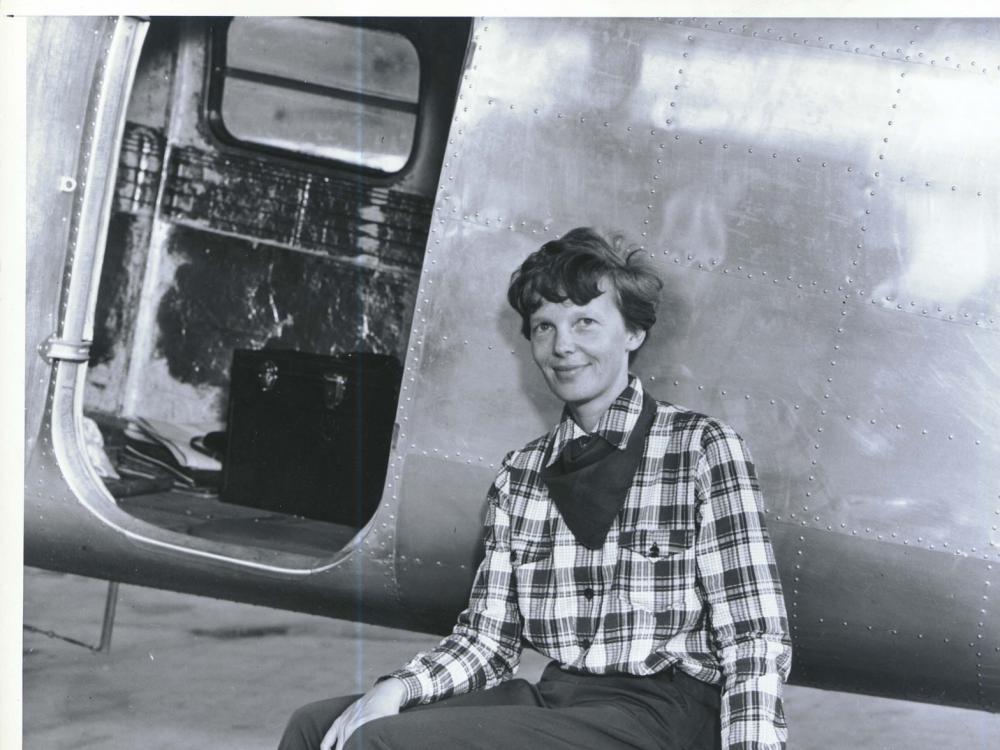This black and white photo captures a young Amelia Earhart, likely in her late 20s or 30s, sitting in front of a grounded metal airplane with visible rivet details across its surface. Amelia, with her short, wavy hair and dark bandana around her neck, is smiling directly at the camera. She is dressed in a checkered, button-up, long-sleeved shirt and dark pants. Behind her is the open door of the aircraft, revealing a black trunk and scattered papers or sundries on the floor. The plane's interior shows a mix of dark panels and lighter sections with black smudges. The setting is on a concrete base, affirming that the plane is not airborne.